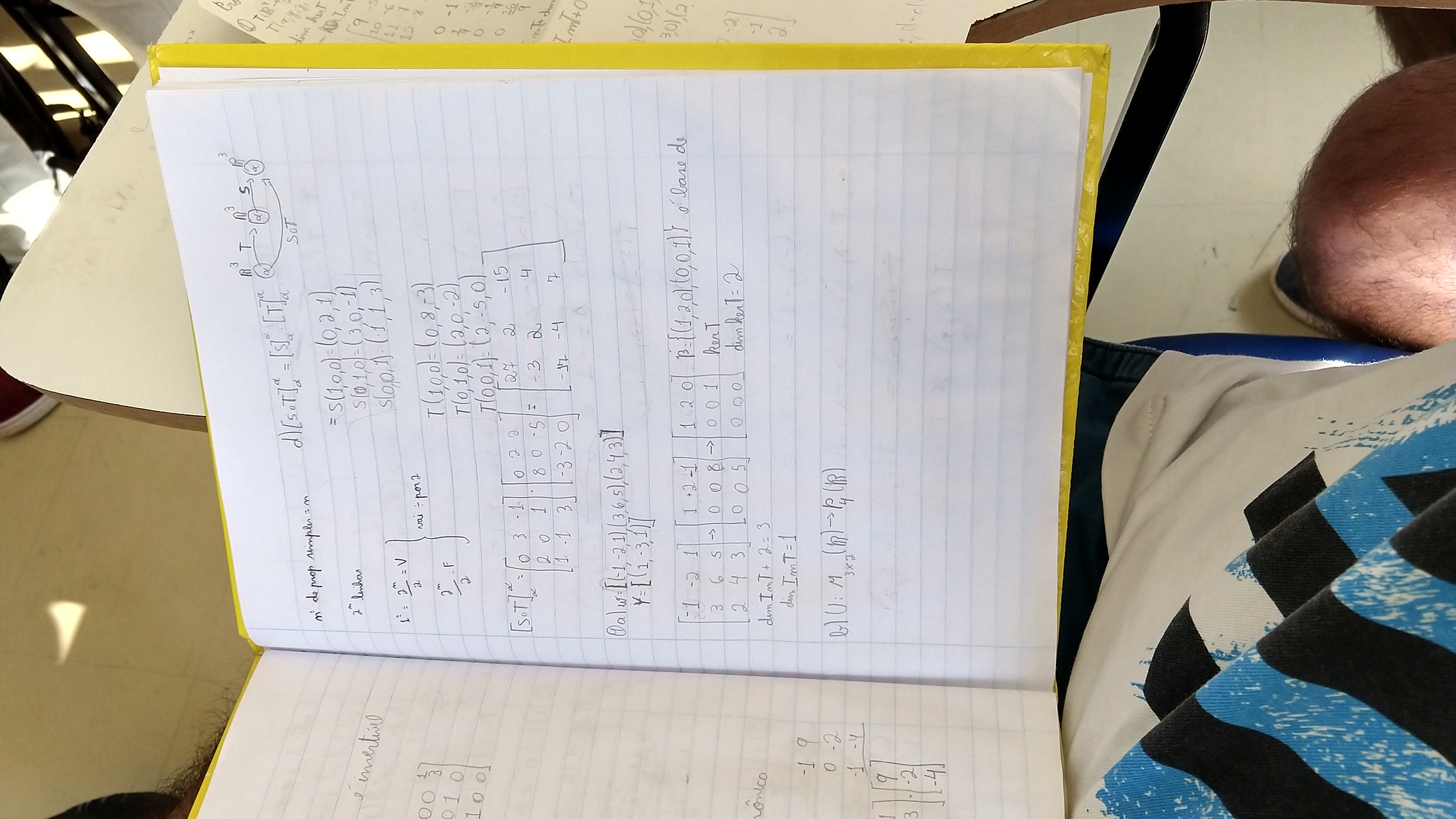The photograph appears to be taken in a bedroom, capturing a diverse yet organized setting atop a bed, part of which is visible in the lower right corner, featuring a white sheet adorned with blue graphic scribbles and black bars. In the upper right corner, a spherical object resembling the top of a baby's head with hair is visible, although its exact nature remains unclear. Dominating the center of the image is an open notebook that could be mistaken for a folder, containing loose-leaf papers on both sides. The left side of the notebook prominently displays a piece of paper filled with pencil writing, potentially math homework, judging by its appearance. Similar pencil markings are noticeable on the lined paper on the right side of the notebook. The lower left corner of the image reveals a white rectangular object situated above a beige carpet. Meanwhile, the upper left corner is marked by the presence of a black mount, providing some contrast to the otherwise light and casual composition.